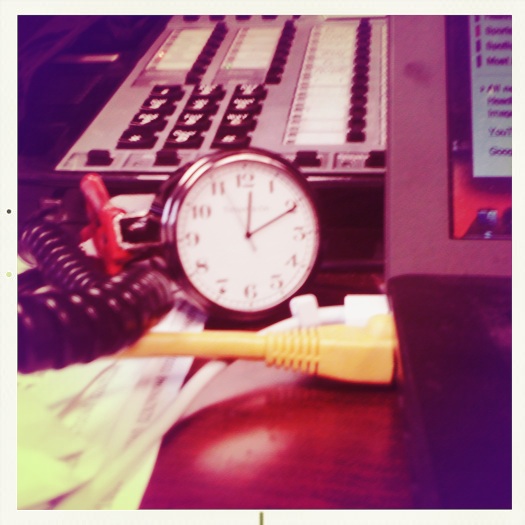This image appears to be an older photograph with somewhat faded or discolored tones. The primary focus is a vintage soundboard, positioned at the top and turned sideways. Sitting directly in front of the soundboard is a classic round wind-up clock, displaying the time as 12:10 and 55 seconds. To the right of the clock, a yellow plug, likely for a phone or Ethernet connection, is inserted into a box. A notable feature is a black rubber spiral cord emerging from the left side of the setup, which curls around and extends downward. All of these items are placed on a desk made of rich, red cherry wood.